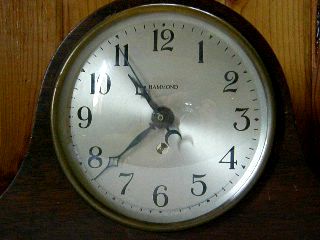This close-up image features a traditional mantel clock set into a beautifully carved wooden frame, showcasing its central design. The clock, rich in character, is embedded in brown wood with finely finished edges, which are not fully visible in the image. The clock's face is encircled by a polished brass ring, adding an elegant contrast to the white background where sleek, traditional numerals denote the hours. Above the center of the clock’s face, a logo is present, though its details are indistinguishable. The time displayed is approximately 10:42. The backdrop of the image is a lighter tan-colored wooden wall, enhancing the darker hue of the mantel clock and adding a rustic charm to the overall composition.